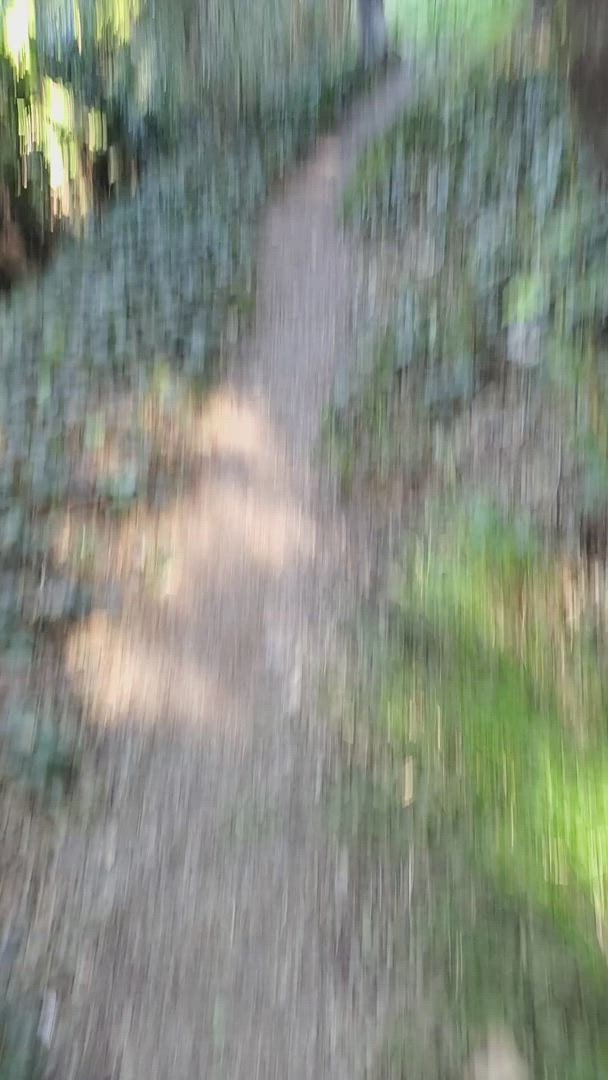A daytime outdoor photograph depicting a scene overwhelmed by extreme blurriness, rendering specific details indistinguishable. On the left side, subtle hints of sunlight illuminate the upper corner, casting a faint glow. Below, a row of indistinct green hues suggests the presence of bushes or vines extending from the bottom center to the upper background. In the middle ground, a brown dirt path meanders through the scene, bordered on its right by patches of darker green, possibly representing more dense foliage or vines. Despite the overall lack of clarity, the image hints at a natural, rustic setting bathed in daylight.